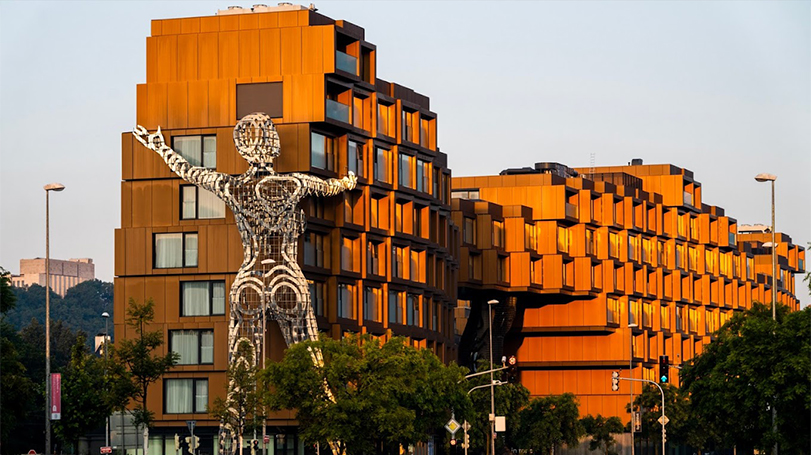The photograph captures a modern, multi-tiered, brown building featuring a unique architectural design with various columns and blocks projecting at different angles. The building exudes a gold-orange hue, contributing to its futuristic appearance. On the middle left of the image, slightly distanced from the main structure, there's a smaller, light tan building. Dominating the foreground is a tall, silver lamppost extending up, crowned with a large, prominent light fixture. 

In the center-left section, a striking steel sculpture designed to resemble an outline of a woman's body hugs the building, almost reaching its top. This art display, with its metal frames and shiny gold plates, adds to the building's contemporary aesthetic. The image also includes green trees, both in the background and the bottom right corner, enhancing the natural element of the scene. Streetlights, signs, and traffic lights (sometimes referred to as "robots") populate the foreground, grounding this architectural marvel in its urban environment. The sky above is a dark gray, providing a moody contrast to the vibrant structures below.